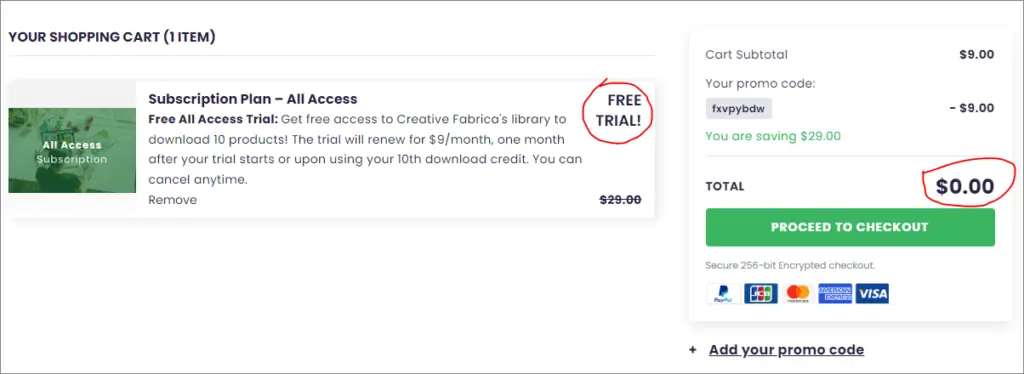The image features the shopping cart section of a shopping app. In the upper left corner, the heading reads "Your Shopping Cart," indicating one item. The item listed is a subscription plan for an All-Access Free Trial. Key details have been highlighted using a digital red marker. The "Free Trial" text and the price "$0.00" in the item's description are circled, emphasizing the trial's cost-free benefit. Notably, the regular price of $29.00 has a strikethrough, highlighting that the trial is free.

The cart subtotal displays as $9.00, but a promo code "FXBPYBDW" has been applied, deducting the $9.00 total. A green note underneath states, "You are saving $29," reinforcing the benefit of the discount. The final total is marked as "$0.00," circled prominently in red. Below this, there’s a green button labeled "Proceed to Checkout."

Icons for various payment options, including PayPal, MasterCard, Visa, American Express, and an unrecognized card, are located at the bottom.